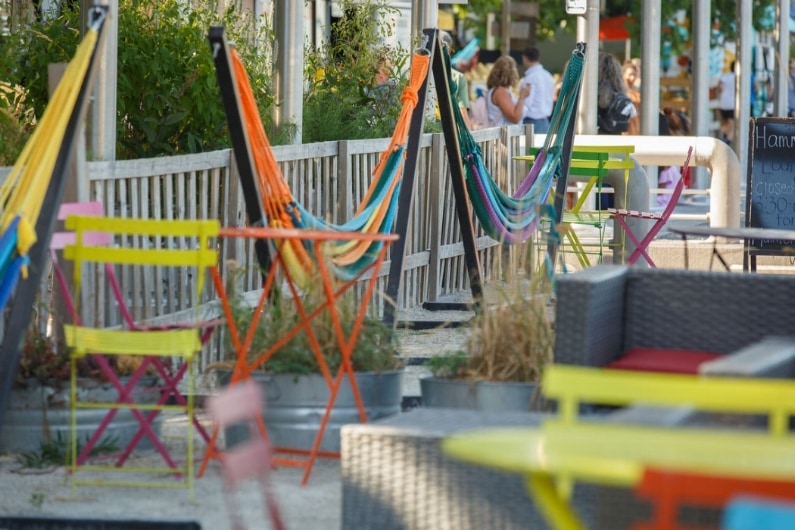This image showcases a vibrant and inviting outdoor lounge area situated in a walkable city, possibly near a beach or a busy pedestrian area. The focal point of the scene features colorful hammocks strung between poles, with hues of blue, purple, yellow, orange, and teal adding to the lively atmosphere. Surrounding the hammocks, there are various seating options, including aluminum or metal chairs and tables painted in vibrant colors, as well as blockier couches or chairs. In the foreground, a small yellow director's chair sits next to a white fence, which is adorned with the colorful hammocks. The area is dotted with metal buckets filled with plants, enhancing the cozy, eclectic vibe. In the background, a couple is seen with the woman resting her hand on the man's shoulder, walking away from the camera, hinting at a leisurely stroll. Beyond them, more pedestrians walk along an alleyway or road lined with shops and restaurants, punctuated by greenery climbing over a wooden fence that separates the seating area from a garden space. The overall setting conveys a lively, bustling, and colorful outdoor retreat.